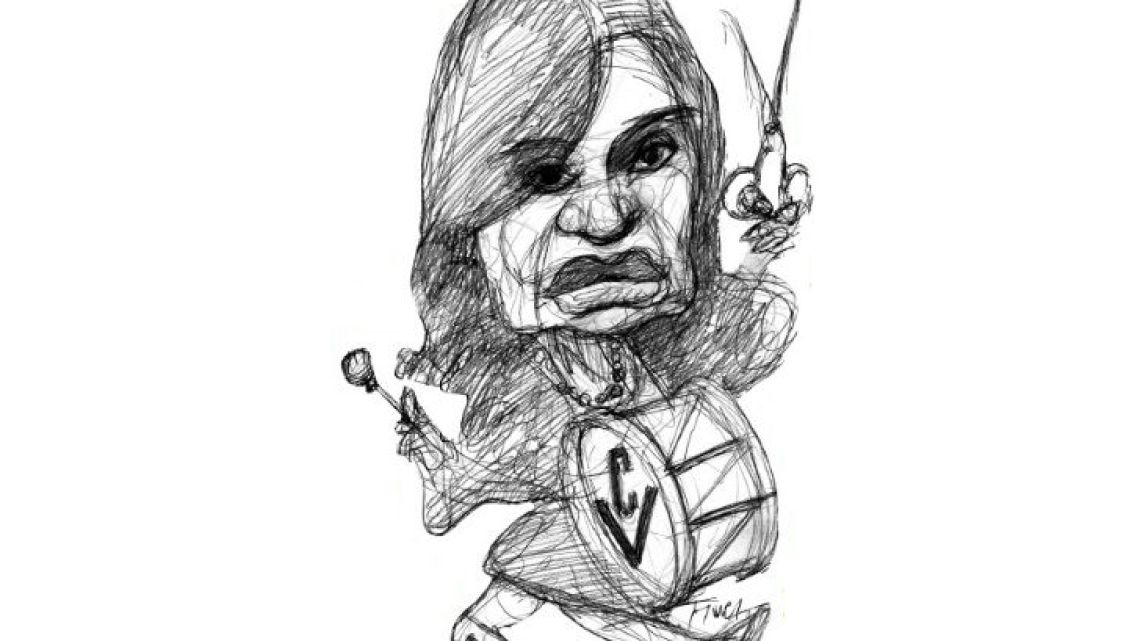The image features a detailed, hand-drawn pencil sketch of a woman occupying nearly the entire frame, set against a completely white background. The artistic style is characterized by scribbly, loose lines. The woman, centered in the image, has exaggerated facial features, including an enlarged nose, nostrils, and oversized lips, while her eyes remain proportionally normal. Her long, wavy hair is adorned with a sideband.

She's dressed in a poofy-sleeved outfit that resembles a dress. Notably, she appears to be walking, with one leg stepping in front of the other. In her right hand, she holds a pair of scissors raised up, and in her left hand, a drumstick. A large drum adorned with the letter 'C' is strapped to her front, positioned in the bottom right of the scene. The entire drawing is rendered in shades of white, black, and gray, giving it a monochromatic appearance.